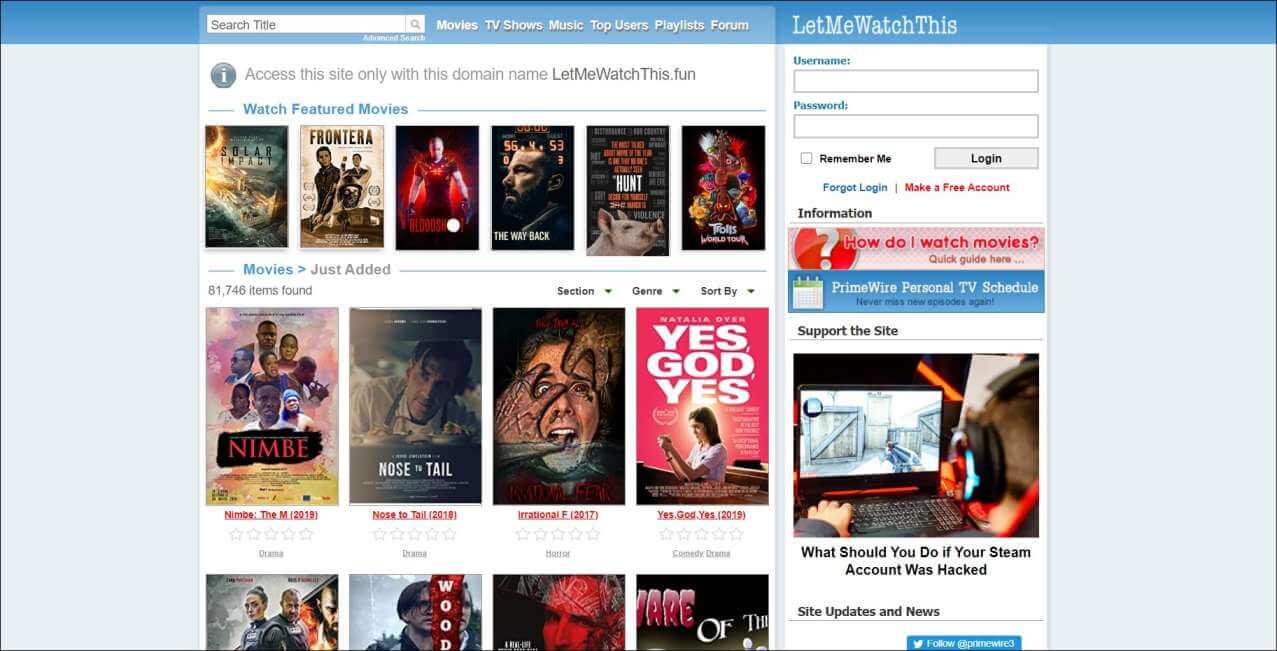A user is interacting with an online streaming platform and exploring various functionalities. The platform offers a variety of options including watching movies, TV shows, listening to music, and accessing user-generated playlists. Users can log in with a username and password, create a free account, and utilize features like 'Remember Me' and 'Forgot Login'. The site also provides a quick guide on how to watch movies, details about Prime Wire, personal TV schedules, and support resources.

In the image, the search results display titles such as "Bay", "Frontera", "Yes, God, Yes", "The Way Back", "Solar Impact", "Trolls World Tour", and "The Hunt". There are also notifications related to site updates and news, including information on what to do if a Steam account is hacked. The platform interface is visually busy with tabs, buttons, and various navigational elements.

This detailed exploration captures a user navigating the rich and multifaceted offerings of an online streaming site, with a particular focus on featured content and user account management options.